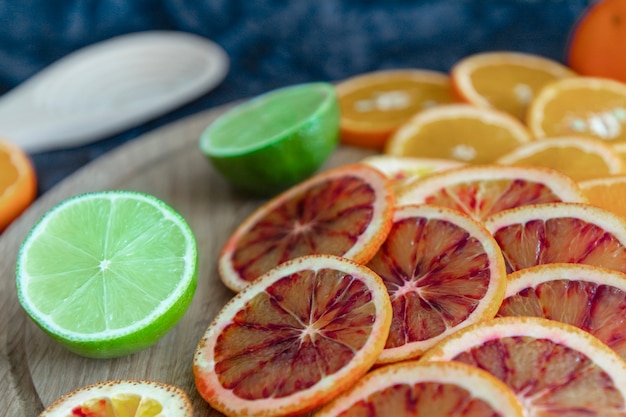This is a detailed color photograph of an assortment of sliced citrus fruits arranged on a circular wooden cutting board with a distinct groove around the edges. The cutting board predominantly occupies the frame, showcasing its pale brown color with a noticeable black grain pattern. On the lower right, several thin slices of blood oranges can be seen, characterized by their vibrant orange and red centers, with a white ring encircling the outer orange skin. To the left, there are two halves of a lime, displaying their green exterior and light green interiors, which are cut side up facing the camera.

In the background, particularly on the upper right, thinly sliced oranges are spread out, revealing at least seven pieces with thin cuts. Adjacent to them on the left is another half of a lime. There is also a whole orange placed in the upper right corner, slightly off the cutting board. An unidentifiable white object, which could be a spoon, is present in the upper left-hand corner. Additionally, a blue object or background element is partially visible on the left side, though it's indistinct and somewhat blurry. The overall arrangement of the fruit and the detailed texture of the wooden board create a visually appealing and intricate display of citrus slices.